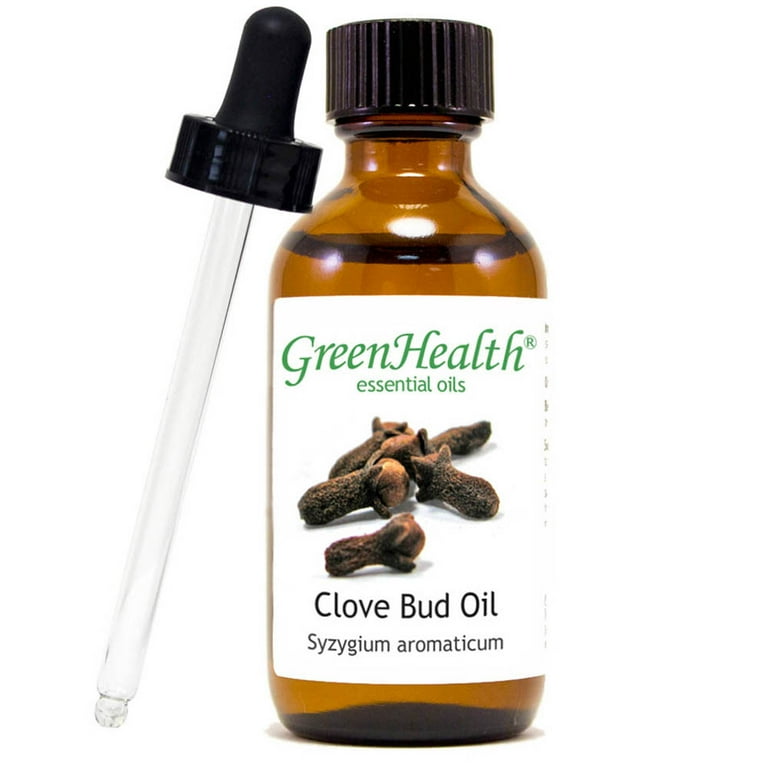The product image is a detailed close-up of a small glass vial with a clear dropper leaning against it, both set against a completely white background. The vial, made of brown glass and fitted with a black cap, contains clove bud essential oil. The label on the vial reads "Green Health Essential Oils" in elegant green cursive on a white background. Below this, a picture of clove buds is prominently displayed, accompanied by the text "Clove Bud Oil" in dark lettering. The scientific name, "Syzygium aromaticum," is also printed on the label. The vial appears nearly full with the amber liquid, which reflects light. The dropper beside the vial has a black lid and is intended for extracting the essential oil.